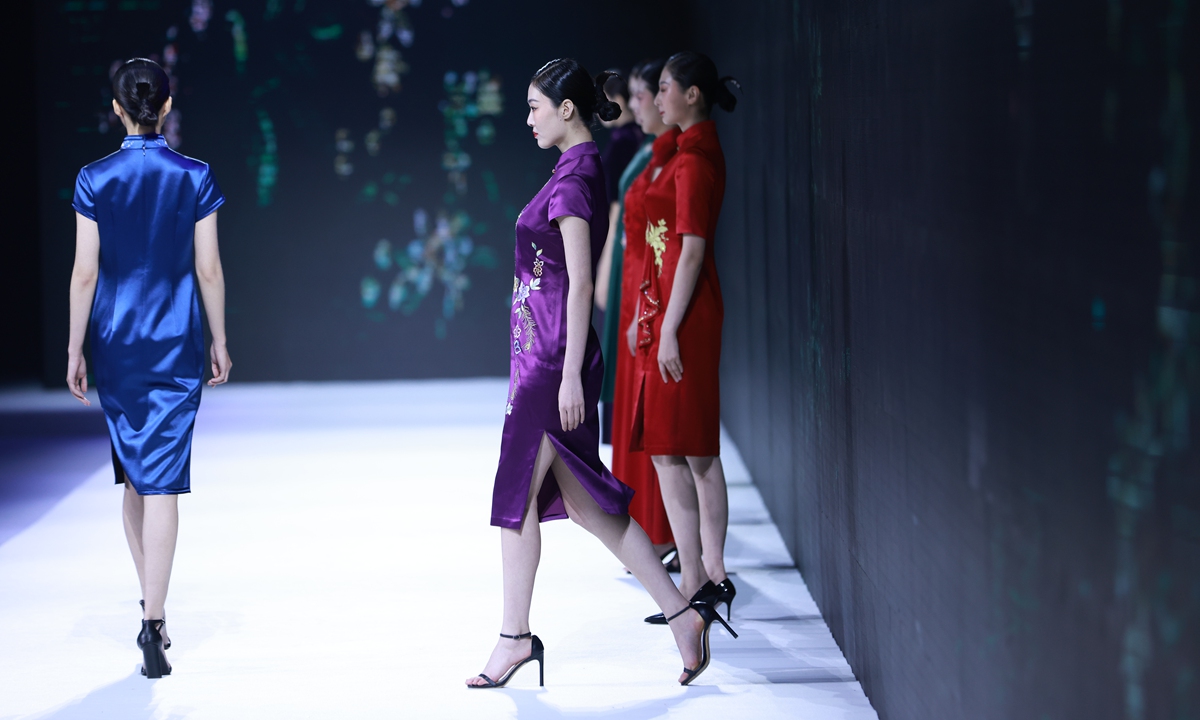In this image of a vibrant fashion runway, the backdrop is a black wall adorned with floral designs. The runway itself is brightly lit and stark white. Dominating the scene is a model in a shiny blue cheongsam dress walking gracefully down the runway. Her dress falls just above her knees and leaves her shoulders bare; she complements her outfit with black high heels and her black hair tied up. Slightly behind her but stepping onto the runway is another model in a silky purple cheongsam featuring a slit on the left side and gold flowery designs. She also wears black high heels with her black hair similarly styled. Waiting behind are several other models: two wearing red cheongsams with gold patterns, one in green, and another in black. All have their black hair tied back, maintaining a cohesive and elegant look as they prepare for their turn under the spotlight.